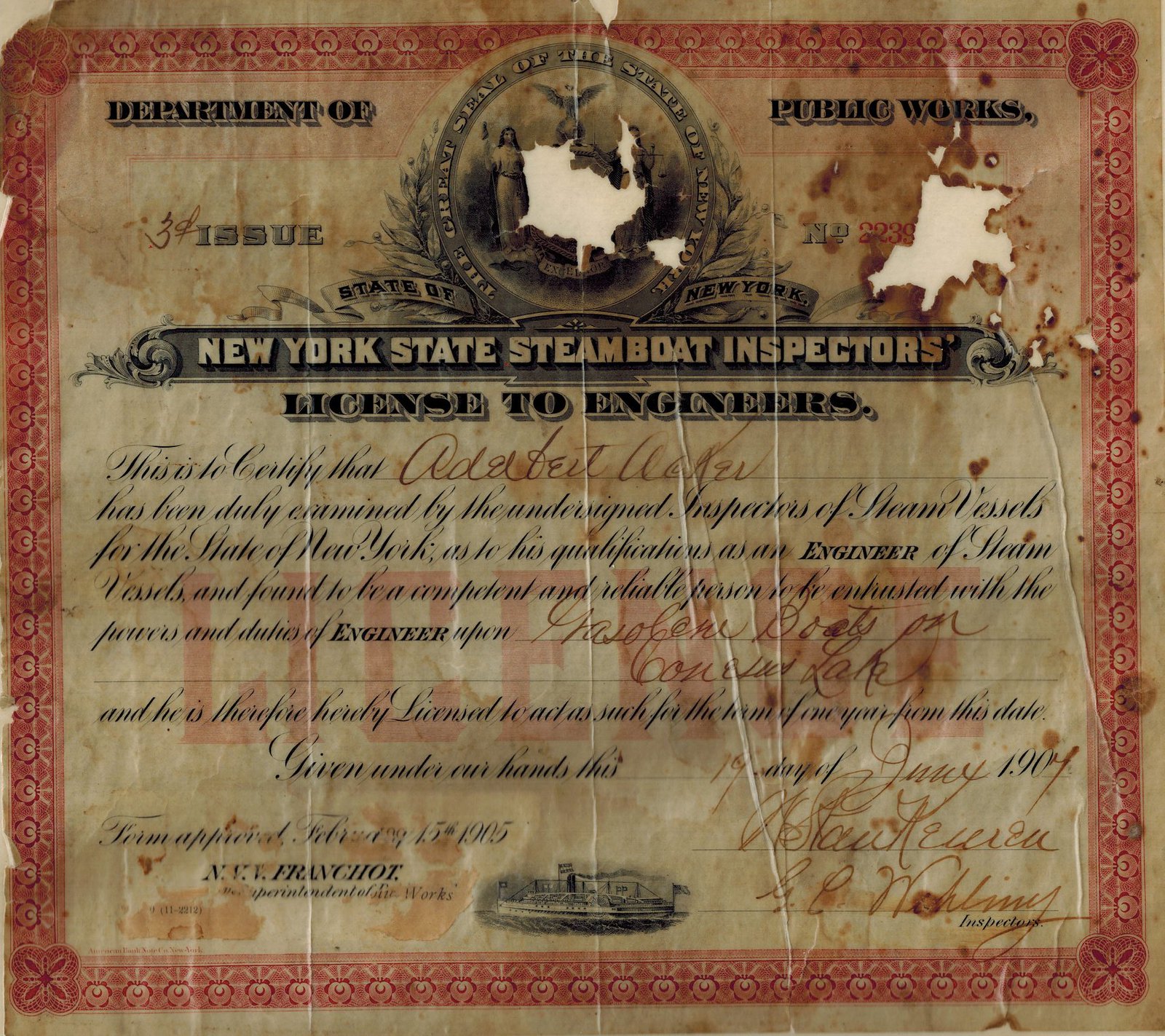This image depicts a very old and worn certificate issued by the New York State Steamboat Inspectors for Engineers, under the Department of Public Works. The document, appearing to be beige-brown with notable black marks and creases, exhibits significant damage, including burns and holes, particularly around the top and center areas. The top banner reads "New York State Steamboat Inspectors, Licensed to Engineers", followed by the words "Department of Public Works" and "Third Issue" on the left. Despite the deterioration, the text 'The Great Seal of the State of New York' and an emblem featuring Native Americans are partially discernible. The certificate certifies that the named individual, though hard to read, has passed the qualifications as an engineer. The main text is in a cursive font, with additional handwritten names and signatures, approximately six in total, dating to February 15th, 1905. The bottom of the document features a printed image of a steamboat.